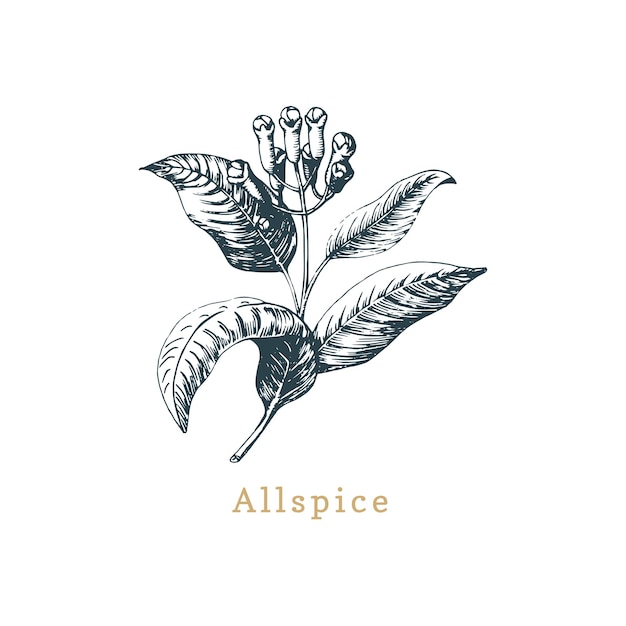The image is a detailed black and white line drawing of an allspice plant, likely from a horticultural book. It features a central stem with four distinct, thick leaves radiating outward. The leaves display intricate details, including curvatures and indentations, with strategic black and white shading to highlight their textures and shadows. The leaves on the left are curved upward, while those on the right are laid out flat. At the top of the stem, there are eight small, cylindrical flower bulbs, presumed to be the seeds of the allspice plant. The background is entirely white, enhancing the focus on the black and white drawing. At the bottom of the image is the word "Allspice" in a light brown or yellow font with a capital 'A', adding a touch of color and identifying the plant.